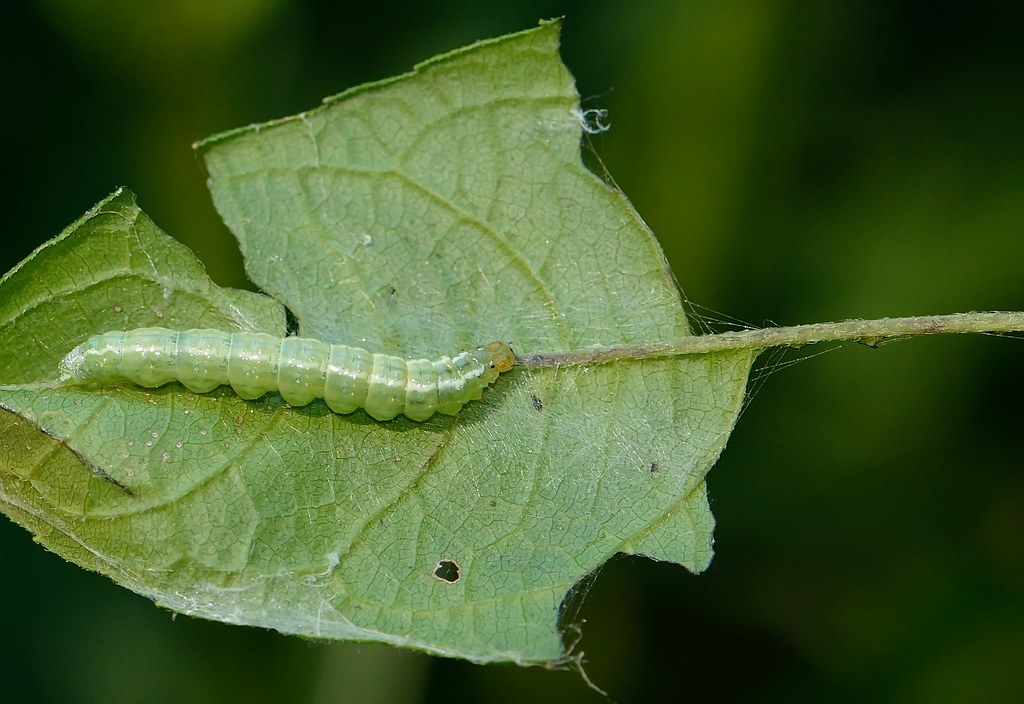A close-up photograph captures a slender, green caterpillar camouflaged on a well-veined, light green leaf with sections eaten away, displaying a network of small holes, tears, and white silk strands presumably from the caterpillar. The caterpillar, with a shiny, almost glistening light green body segmented into twelve parts, is crawling horizontally across the leaf, its position aligned with the main vein and heading towards the stem. It has small, seemingly delicate features, including tiny eyes and a subtle brownish or yellowish head. The backdrop of the image is a blurred green and black, suggesting a forest or leafy area, which contrasts sharply with the crisp detail of the leaf and caterpillar in the foreground. The intricate details of the leaf's veins and the caterpillar's texture highlight its youthful stage before it eventually forms a cocoon. The composition emphasizes the caterpillar's natural camouflage against the vibrant leaf, set in a serene, verdant environment.